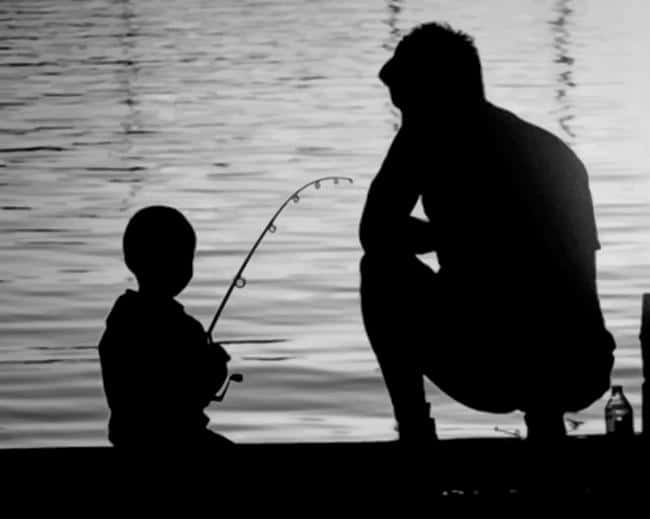In a black-and-white photograph, a serene scene unfolds on a dark, possibly dock-like surface set against a silvery gray expanse of shimmering water. Dominating the right side of the image, a silhouetted man with short hair crouches on his haunches, his left elbow resting on his knee as he looks down contemplatively. He wears shorts with his socks peeking out, adding to the casual, relaxed feel of the scene. Beside him, slightly to his left, a young boy with short hair kneels, engaged in the timeless act of fishing. The boy's fishing rod is clearly silhouetted, its reel handle and metal hoops distinct against the luminous backdrop of the water. The rod is bent at the front, suggesting a catch, capturing a fleeting moment of excitement. Just to the man's right, a clear bottle is faintly discernible on the dark surface, adding a touch of realism to the tranquil setting.